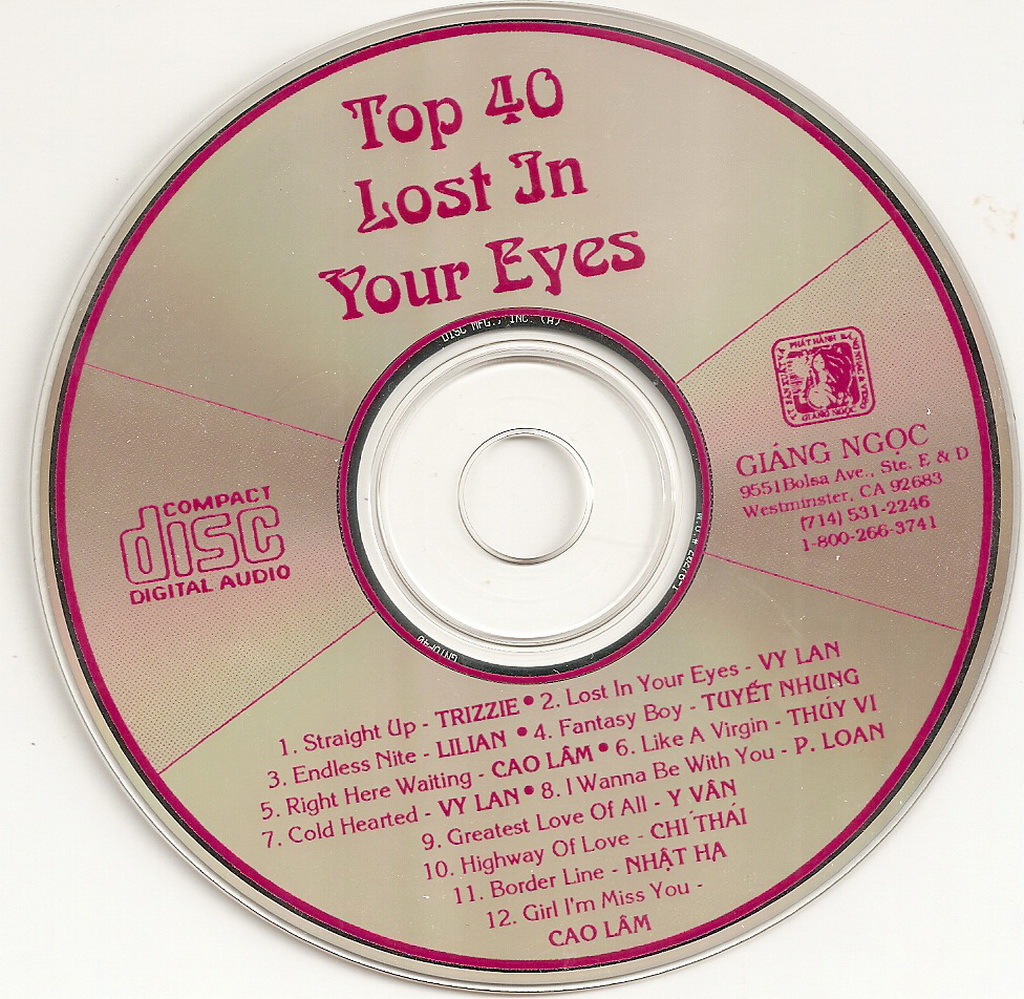This is a large square image with a gray background, though mostly obscured by a very large compact disc dominating the frame. The disc is silver with distinct red writing and a red border along its edge. At the top, the title "Top 40 Lost in Your Eyes" is prominently displayed in red. On the left-hand side, the compact disc features the text "compact disc digital audio." The right-hand side showcases a square logo with the text "Giang Ngoc," which is followed by an address in Westminster, California with the ZIP code 92683, and phone numbers including (714) 531-2246 and a toll-free number 1-800-366-3741. The bottom section of the disc lists 12 song titles, each numbered and centered atop one another. Song titles such as "Straight Up - Trizzy," "Lost in Your Eyes - Vi Lan," and "Girl, I Miss You - Chow Lam" suggest a mix of English titles by artists with Vietnamese or Thai names. The artists contributing to this compilation include Trizzy, Vai Lan, Lilian, Thuyet Nung, Kalam, and Thuy Vy.